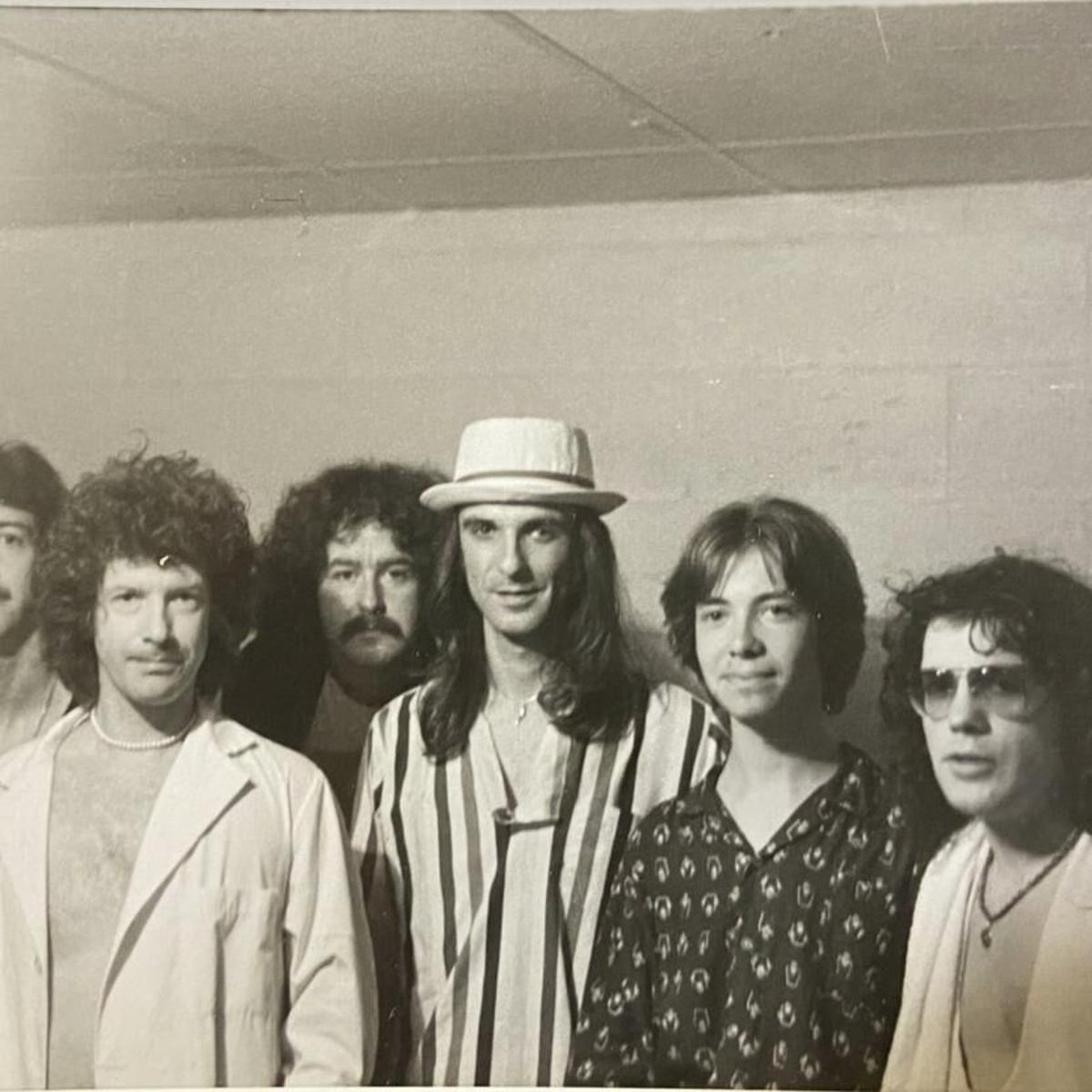This black-and-white photograph, likely taken in the 1970s, features six young men standing against a white cinder block wall with a white drop ceiling overhead. The group has a distinctly retro vibe, reminiscent of 70s rock bands. All the men have long hair, varying from curly to straight styles, and several sport mustaches. Starting from the left, the first man is only partially visible, showing just his eye and some of his straight dark hair. Next to him, a man with straight dark hair parted in the middle wears a dark button-up shirt with a lighter pattern. In the middle of the group, a man with long, straight dark hair dons a white hat with a small ring around it and a striped button-up shirt, with a small light-colored necklace. Standing behind him is a man with very puffy, dark curly hair and a handlebar mustache, whose face is the only part visible. The next individual, with curly dark hair and a thin mustache, wears an open button-up shirt and a white bead necklace. The final man on the far right has curly black hair, sunglasses, an open white shirt revealing a bare chest, and a necklace with a small pendant. Together, their eclectic appearance and attire evoke the quintessential look of a vintage rock ensemble.